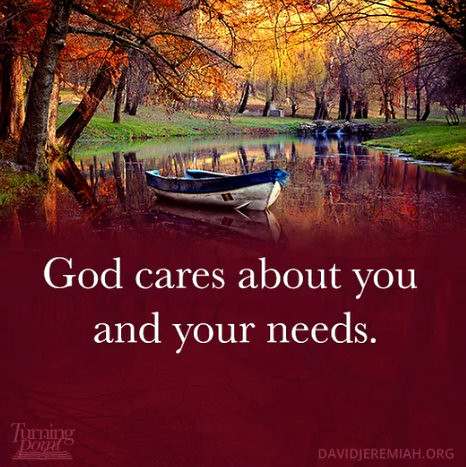This square image depicts a serene yet striking scene of a small body of water, possibly a pond or narrow creek, with unusual red-colored water. A white and blue canoe is positioned centrally on the vivid red water, which occupies the lower two-thirds of the image. The backdrop features a beautiful array of trees adorned with autumn foliage in warm hues of orange and yellow, vividly reflecting the golden light, likely from a setting sun. Flanking the water's edges is lush green grass that gently slopes upwards, framing the basin of the water. Across the center of the image, bold white text reads, “God cares about you and your needs.” Additionally, in the lower left-hand corner, slightly obscured by the dark red water, is the text “Turning Point” in a lighter red font, while the lower right-hand corner displays "DAVIDJEREMIAH.ORG" in all capital letters.